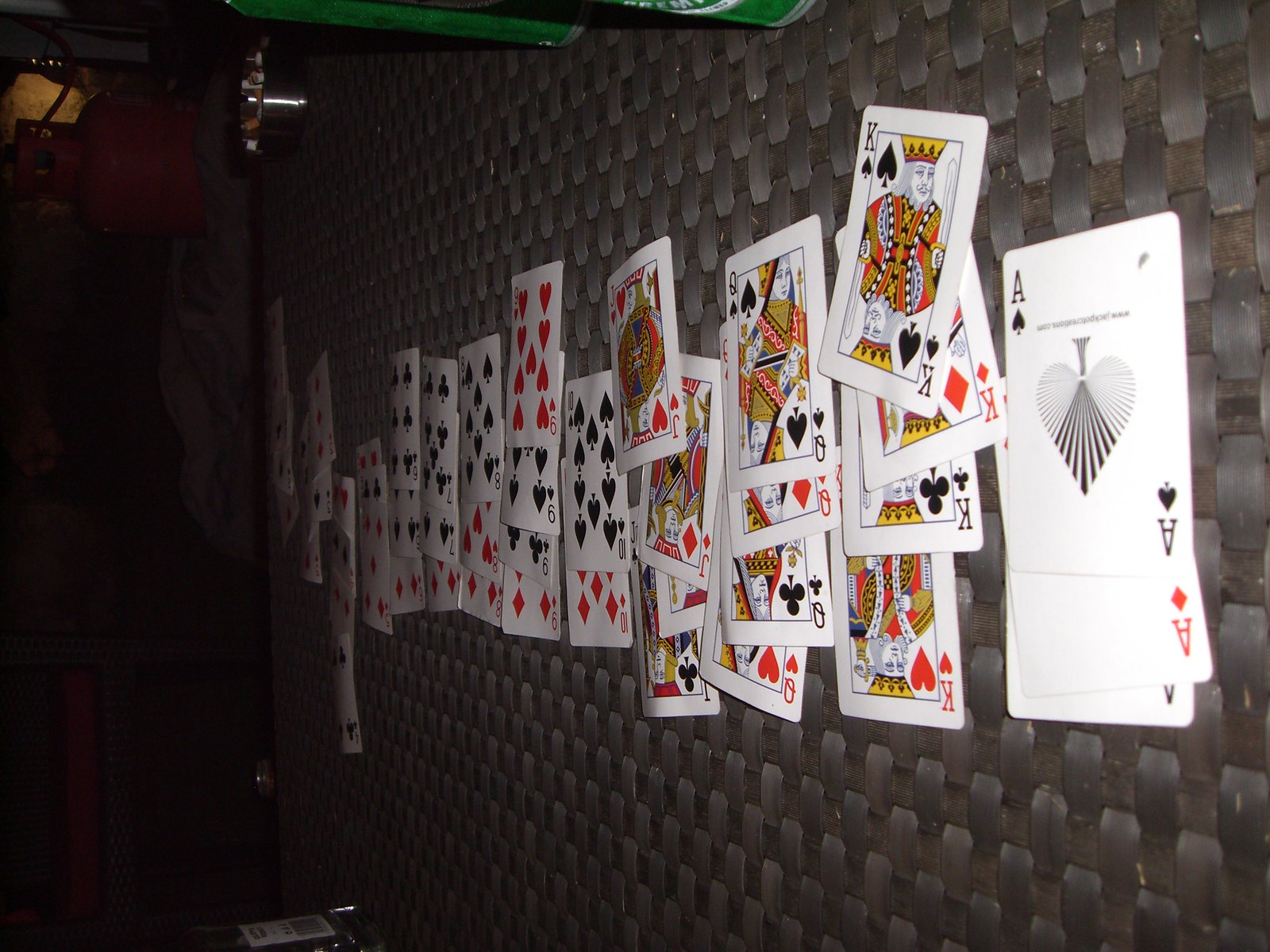Array of playing cards meticulously arranged on a tabletop: On the right side, the Ace of Diamonds is accompanied by another Ace below it, followed by a descending sequence of Kings, Queens, Jacks, 10s, and so forth. Additionally, black heart symbols accentuate the layout. Green beer bottles sit upright atop the table, suggesting the photo is taken from a sideways perspective. This elaborate arrangement combines the elements of gaming and leisure in a vibrant display of colors and patterns.